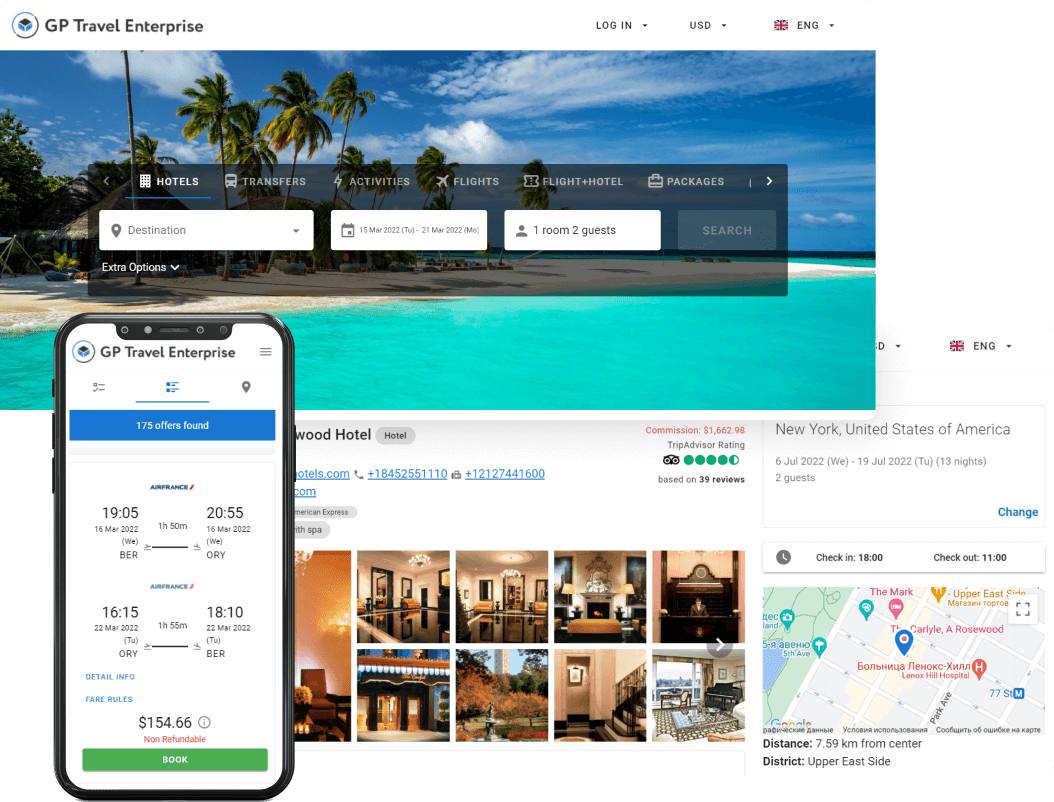The image features the JP Travel and Surprise webpage interface. Dominating the top left of the image, in black text, is the site logo "JP Travel and Surprise." On the top right, several navigation options are displayed, including tabs for Login, currency selection (USD), and a language setting currently set to English, represented by a blue, red, and white UK flag.

The user interface is structured with a transparent black overlay that hosts a comprehensive search filter segmented into three distinct boxes: Destination, Check-in/Check-out Dates, and Number of Guests/Rooms. To the right of these filters is a Search button. Above the search filter, several tabs such as Hotel, Transfer, Activities, Flight, Flight+Hotel, and Packages are listed, with the "Hotel" tab highlighted by a blue underline on its left side.

The background of the interface showcases a picturesque beachfront scene. This vivid image includes a clear blue ocean, brown sandy beach, and tall green trees, accented by people enjoying the scenery. Above, the sky is a tranquil blue with scattered white clouds.

Toward the bottom left of the image, there's a depiction of a smartphone displaying the JP Travel and Surprise app. Here, the app indicates "175 offers found" with a highlighted option priced at $154.66, marked as non-refundable. Adjacent to this price, a prominent blue "Book" button invites action. Flanking the phone to the right, there’s an image depicting an example hotel and its TripAdvisor rating, notably 4.5 stars.

In the bottom right corner, a detailed map highlights critical geographical information about a location in New York, United States of America. It states the area is 7.59 kilometers from the city center, specifically located in the Upper East Side district.